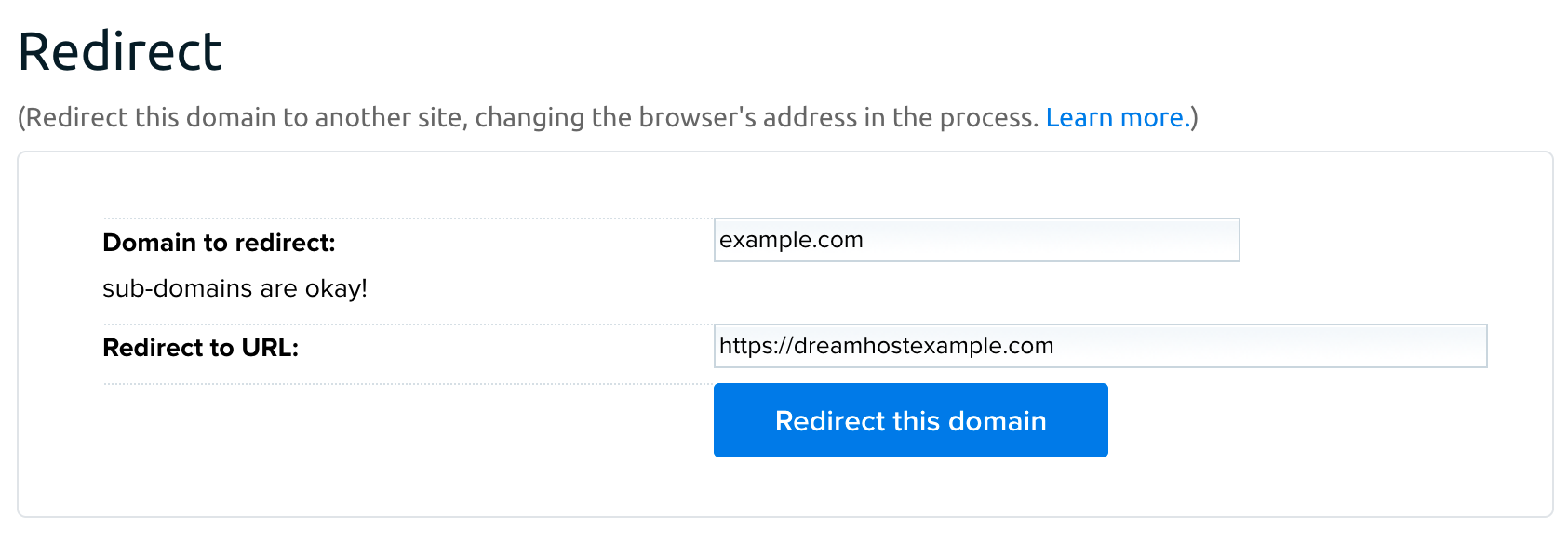This image captures a section of a web page detailing a domain redirection process. At the top, the word "Redirect" is prominently displayed in large black letters. Below it, a short description in gray reads, "Redirect this domain to another site, changing the browser's address in the process (Learn more)." The phrase "Learn more" is hyperlinked in blue.

Beneath the description, there is a rectangular input box with a thin gray border, elongated in landscape orientation, approximately three to four times wider than it is tall. Just below this box and set against a white background, the text "Domain to redirect" is bolded, followed by the reassurance, "Subdomains are okay!" To the right of this text, there is another rectangular input box, white with a blue top, containing the placeholder text "example.com."

The section is further divided by a thin gray line. Below this divider, "Redirect to URL" is written in bold letters, followed by another input box of similar design to the first, containing "https://dreamhotpostexample.com." Finally, at the bottom of the section, a long blue button with white text bears the command, "Redirect this domain."